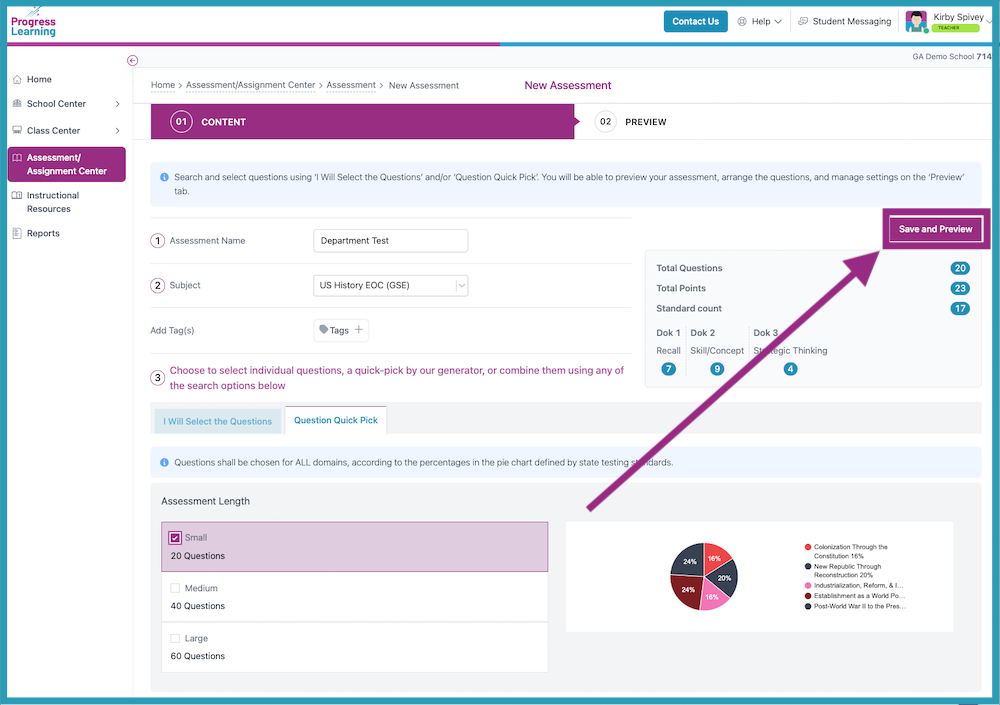**Detailed Caption:**

The image displays a user interface titled "Progress Learning" with "Progress" in purple and "Learning" in blue, each word set on separate lines. A diagonal gradient line transitions from pink to blue, running from the left to the right of the interface. At the upper right corner, the option "Contact Us" is displayed, accompanied by a help section with a dropdown box, student messaging features, and a login status indicating the user is Kirby Spivey, a teacher.

Below the "Progress Learning" title, there’s a vertical navigation column on the left side, featuring several buttons: Home, School Center (with a clickable arrow for more information), Class Center (similarly expandable), Assessment Center (highlighted in purple to indicate the current view), Instructional Resources, and Reports. 

On the main workspace to the right, a breadcrumb trail indicates the user is at "Home > Assessment > Assessment > New Assessment" with various clickable subcategories. Below this, a section labeled "01 Content" in purple and "02 Preview" in blue is visible. It prompts the user to "Search and select questions," allowing for the selection of questions via a "Quick Pick" tool. 

Here, assessment details can be entered; currently, the assessment is named "Apartment Test," indicated for the subject "U.S. History, EOC, JSE." There’s an option to tag individuals, visible on the right, along with boxes displaying the total number of questions, points, and standard counts. A "Save and Preview" button in purple is located above with an arrow pointing to it.

Further down, two tabs are visible where one can select questions using the "Quick Pick" tool. The highlighted length setting is "Small" for 20 questions, with additional settings for 40 (Medium) and 60 (Large) questions. A pie chart graphically represents the distribution of questions by historical periods: Colonization, New Republic, Industrialization, Establishment, and Post-World War II.